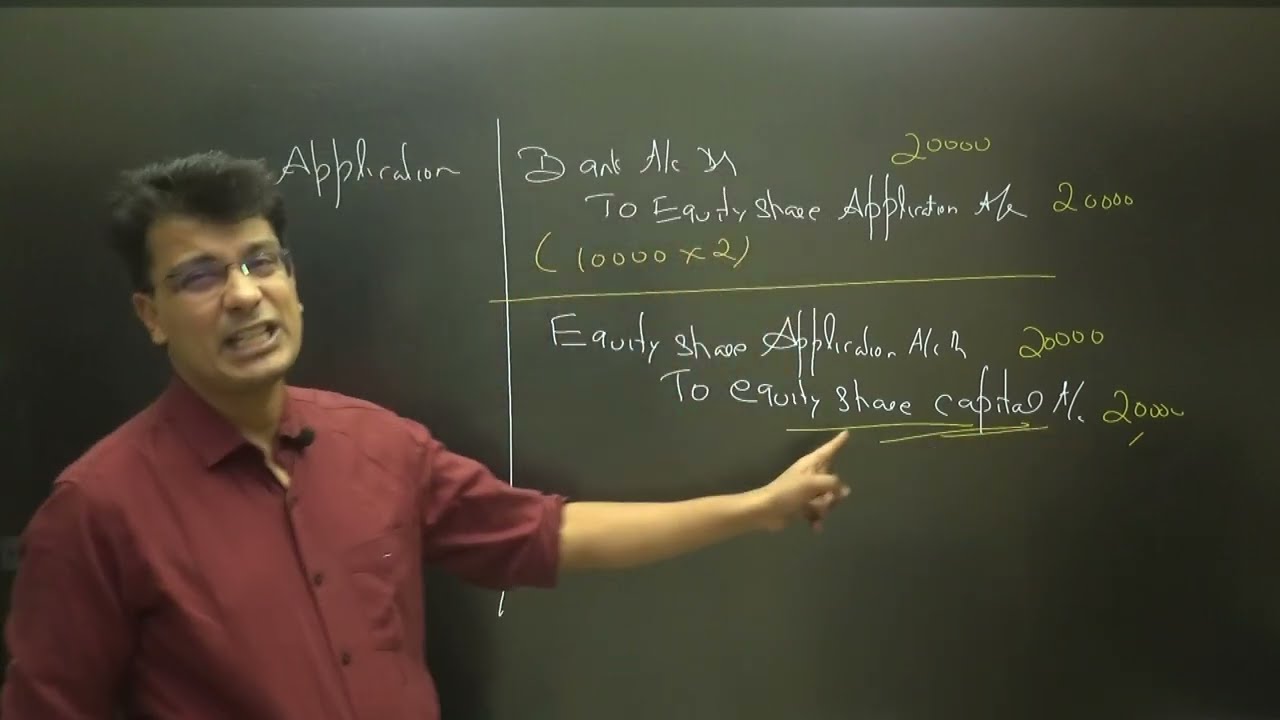The image depicts a teacher with medium brown skin, framed by short, voluminous black hair, wearing frameless glasses and a maroon button-up shirt with the sleeves rolled up to his elbows. He stands slightly to the left, facing the camera and gesturing toward a dark gray or greenish-blackboard with his right hand. His mouth is midway through speaking, revealing tightly clenched teeth.

The blackboard, marked by both horizontal and vertical yellow and white lines, is covered in text written primarily in white and yellow chalk. The legible portions of the text include phrases like "application," "bank to equity share application," and "equity share capital." The board also features numerical notations such as "1,000 x 2" and "20,000," which are emphasized with underlying yellow squiggles. The content appears somewhat messy and in cursive, making it difficult to read clearly. The teacher seems to be explaining the lower section of the text, pointing toward it as he speaks.

Additionally, a small black microphone can be seen clipped to his collar, suggesting he might be addressing a larger audience or recording a lecture.